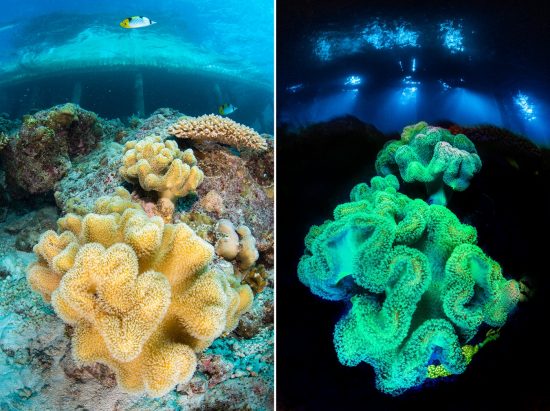The given image is a collage of two underwater photographs, one on the left and one on the right, showcasing identical scenes in different lighting conditions. Both photographs depict an underwater setting featuring a king statue with surrounding marine life. In the left image, under normal lighting, there is a prominent yellow sea organism in the foreground, with similar organisms spotted behind it. Two fishes, colored yellow and white, swim nearby. Behind the fishes is a large metal structure submerged in water, accompanied by visible sea rocks. The right image, taken with a luminescence effect, now shows the previously yellow organisms glowing light green, and blue light is emanating from the metal structure. The water appears darker at the top, emphasizing the luminescent effect and creating a captivating contrast with the left photograph.